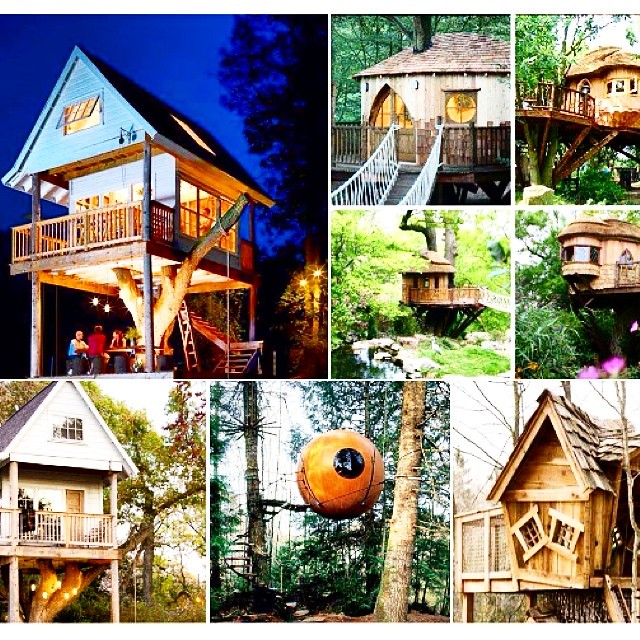This is a color photo collage of eight distinct tree houses, each showcasing a different design and aesthetic. Set against a dark blue sky with scattered trees, the collage features diverse structures, including one in the top left resembling a conventional house perched on a tree with an upper level accessible by a staircase. This house has a balcony and a window on its top level. In the middle towards the bottom, there is a completely round, spherical tree house with a spiral staircase leading up to it, suspended between trees. Two of the tree houses have the tree trunks extending through their bases, each featuring a built-on deck at the front. Some of the tree houses are accessed by rope stairs. The tree houses come in various colors and shapes, ranging from traditional house-like designs to unique round forms. This collage may serve as a conceptual brainstorm for potential designs, either for personal inspiration or as offerings from a builder's portfolio.